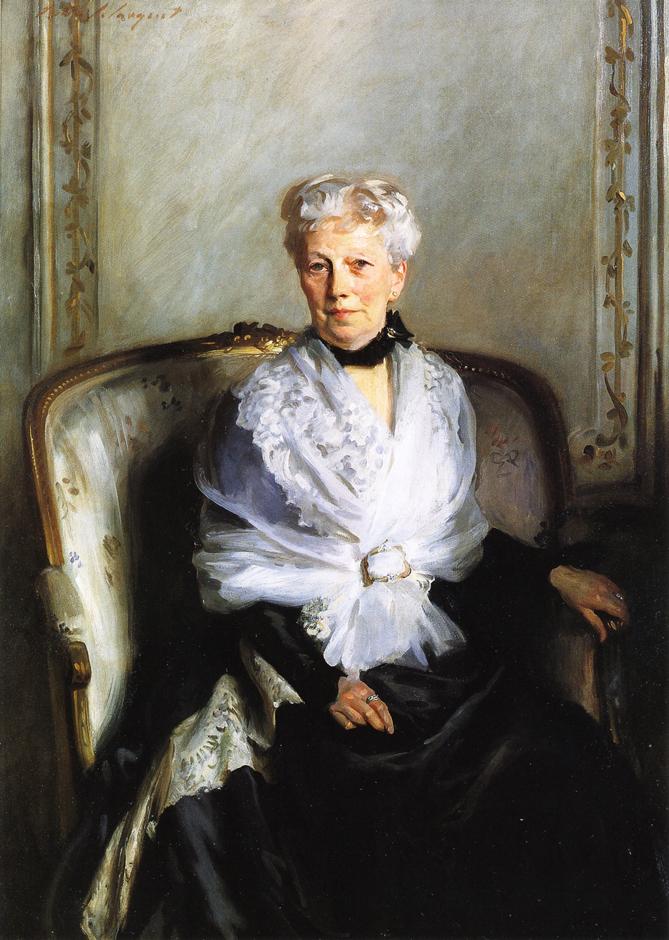A highly detailed, life-like portrait painting of an older woman, showcasing remarkable skill. The woman, who has short, white, curly hair and dark brown eyes, sits facing slightly forward in a very wide-backed, Victorian-style chair with gold or copper trimmings. Her light peachy skin exhibits a slight redness on her cheeks, adding to her stately presence. She dons a black dress with dramatic, dark tones draped elegantly over her lap. A white, lacy, see-through scarf wraps around her shoulders, fastened at the front with a gold brooch. She also wears a black band around her neck. Her hands are positioned with grace—one resting on the armrest and the other downwards, adorned with silver rings. The background features a light gray wall embellished with a square outline containing floral patterns and gold trim, enhancing the painting’s vivid and beige-dominated overtone. The overall composition is both vivid and steady, balancing wildness in the brushstrokes with meticulous detail, capturing the essence of the elderly lady with tremendous skill.